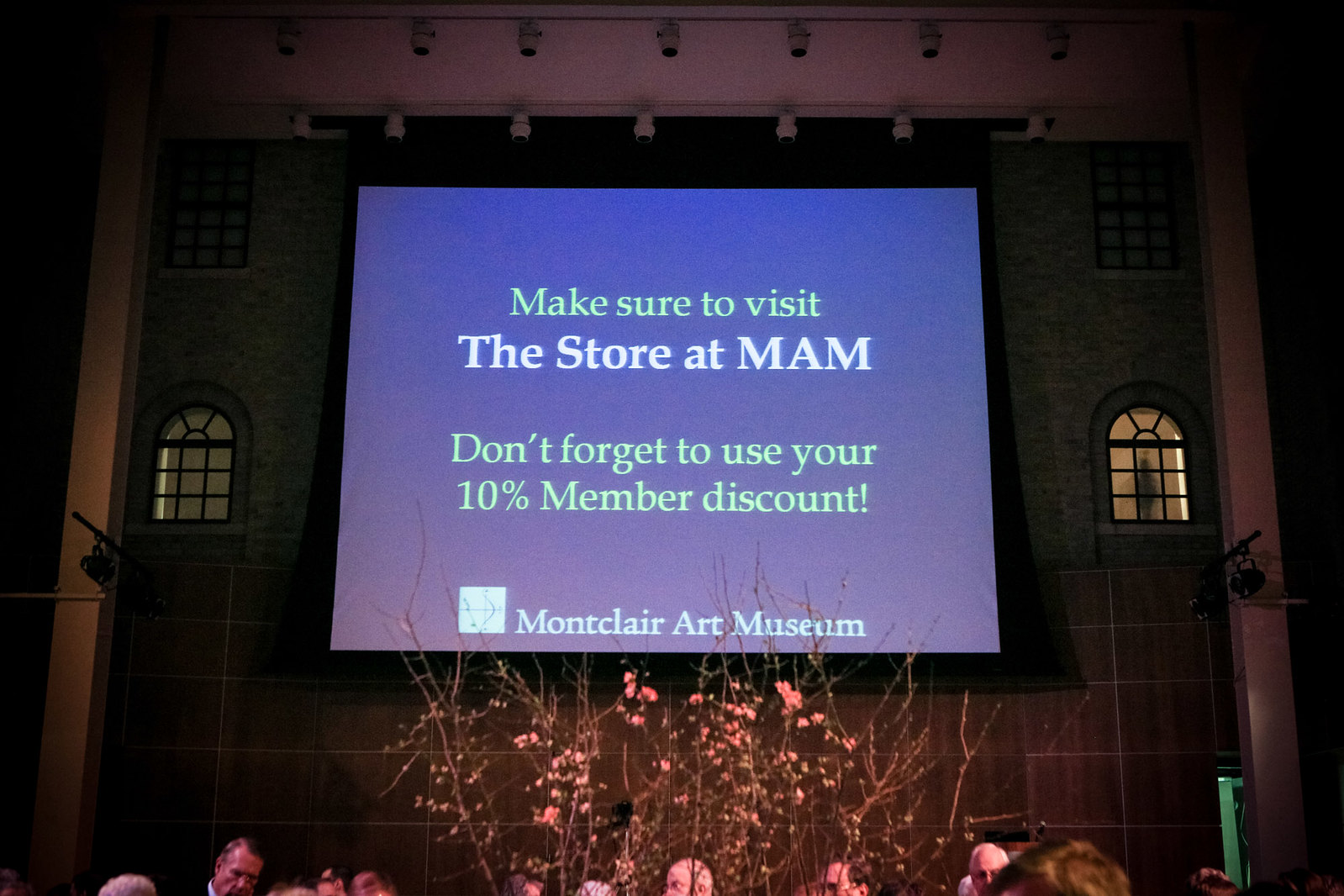A vibrant sign stands prominently on stage, resembling one that might typically be affixed to the exterior of a building. The sign's background features a gradient with a blend of rich blue at the top, seamlessly transitioning into a deep purple at the bottom. The text on the sign encourages visitors to "Make sure to visit The Store at MAM; don't forget to use your 10% member discount!" An exclamation point underscores the importance of the message. At the bottom of the sign, "Montclair Art Museum" is written in a complementary pastel green, juxtaposed against the bold white letters of "The Store at MAM."

In the bottom left corner, adjacent to the museum's name, there is a small square. Flanking the sign are two arch-shaped windows, one on each side, through which the warm glow of interior lights can be seen, suggesting activity and welcoming warmth inside.